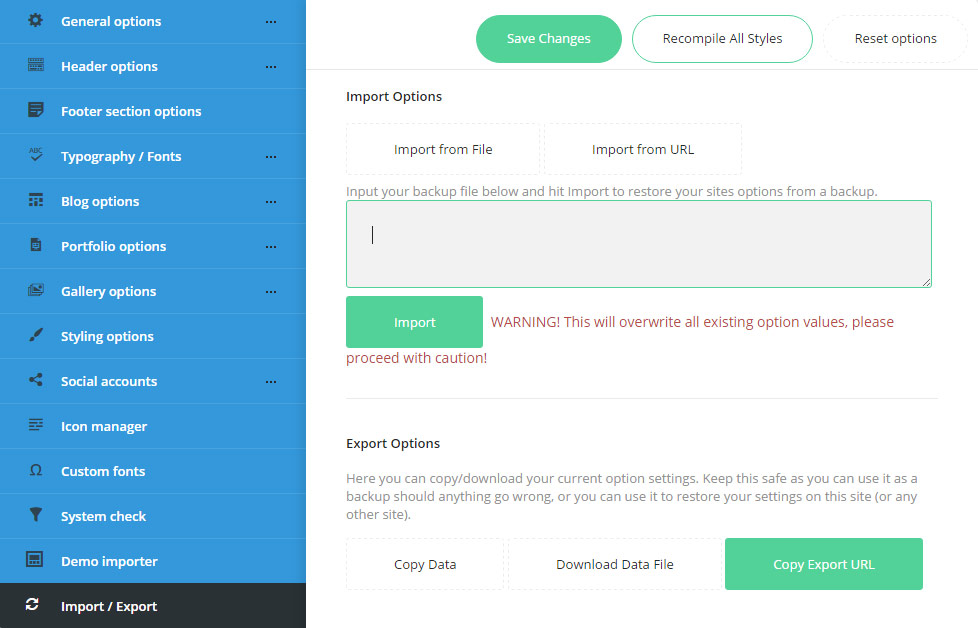The image displays a snippet of a website's user interface, specifically a settings or options panel. On the left side of the image is a tall, vertical blue rectangle with white text listing various menu items: "General Options," "Headers," "Footer," "Section Options," "Typography," "Fonts," "Blog Options," "Portfolio Options," "Gallery Options," "Styling Options," "Social Accounts," "Icon Manager," "Custom Font," "System Stack," "Demo Importer," "Importer," and "Exporter." Among these, the "Exporter" option is highlighted in black, indicating it is currently selected.

To the right, on a white background, the heading "Import Options" is displayed prominently. Below this heading, there is a green "Save Changes" button and a white "Recompile All Styles" button with a green outline. Adjacent to these is a "Reset Options" button featuring black text on a white background. 

Further down under "Import Options," users can choose to "Import from File" or "Import from URL." The interface prompts users to input their backup file into a data field edged in green and provides a green "Import" button for initiating the process. A cautionary warning in red text states: "Warning, this will override all existing option values. Please proceed with caution."

Below the import section is the "Export Options" heading. It provides instructions for copying or downloading current option settings to keep them safe as a backup. Users can then restore these settings on the current site or a different one. The interface includes buttons for "Copy Data," "Download File," and "Copy Export URL."